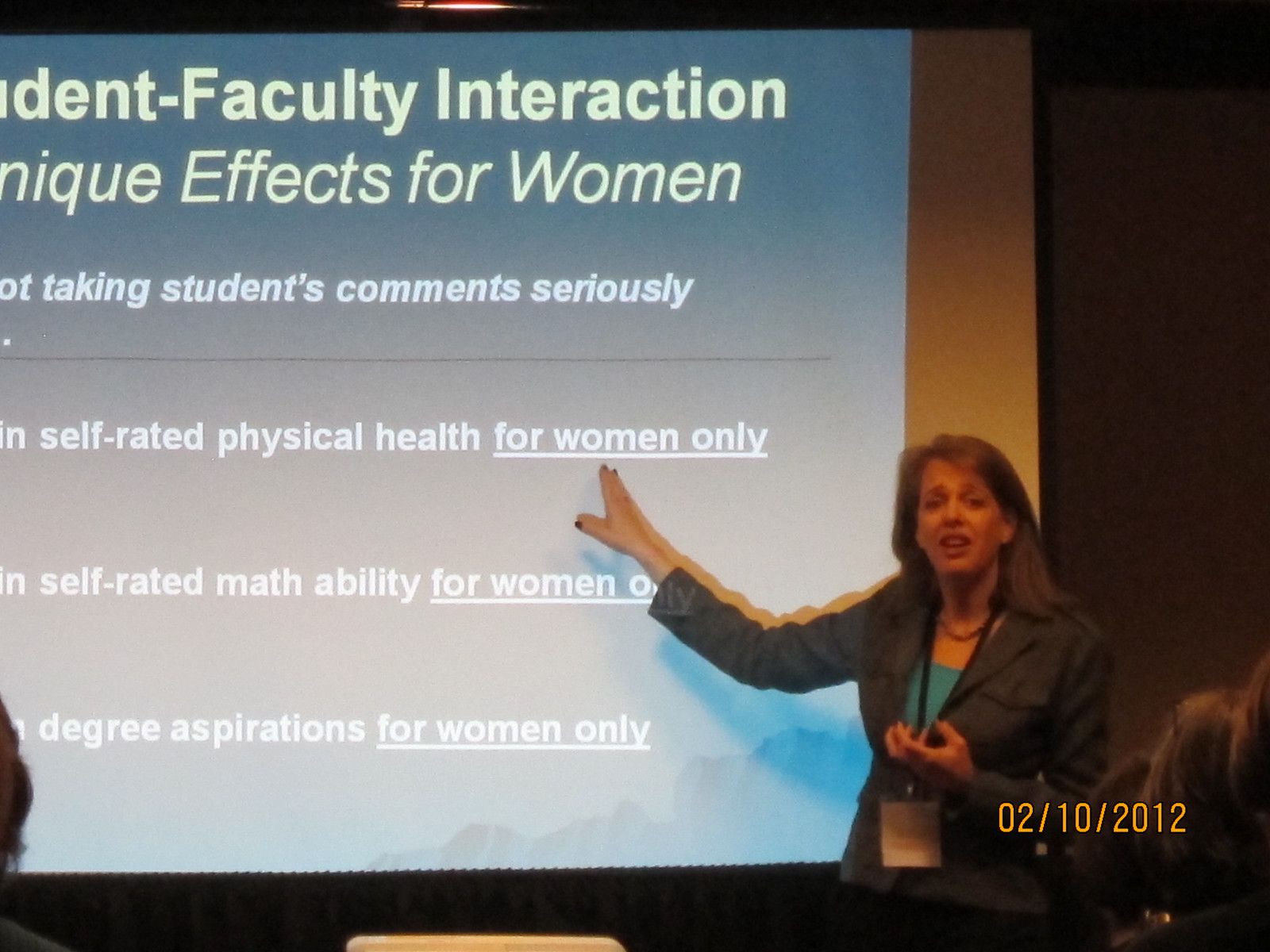In this image, we see a woman presenting a PowerPoint slide on the topic of "Faculty Interaction Effects for Women." The PowerPoint itself has a blue background, and although some of the text is partially cut off, it includes phrases such as "Self-rated Physical Health for Women Only," "Self-rated Math Ability for Women Only," and "Degrees and Aspirations for Women Only." The presenter appears to be around 40 years old, with brown hair. She is dressed in a gray vest suit jacket over a blue undershirt and wears a lanyard. In the audience, visible in the bottom left and right-hand corners of the image, several people are attentively listening to her presentation. Additionally, there is a yellow text watermark in the bottom left-hand corner that reads "02-10-2012," indicating the date of the presentation.